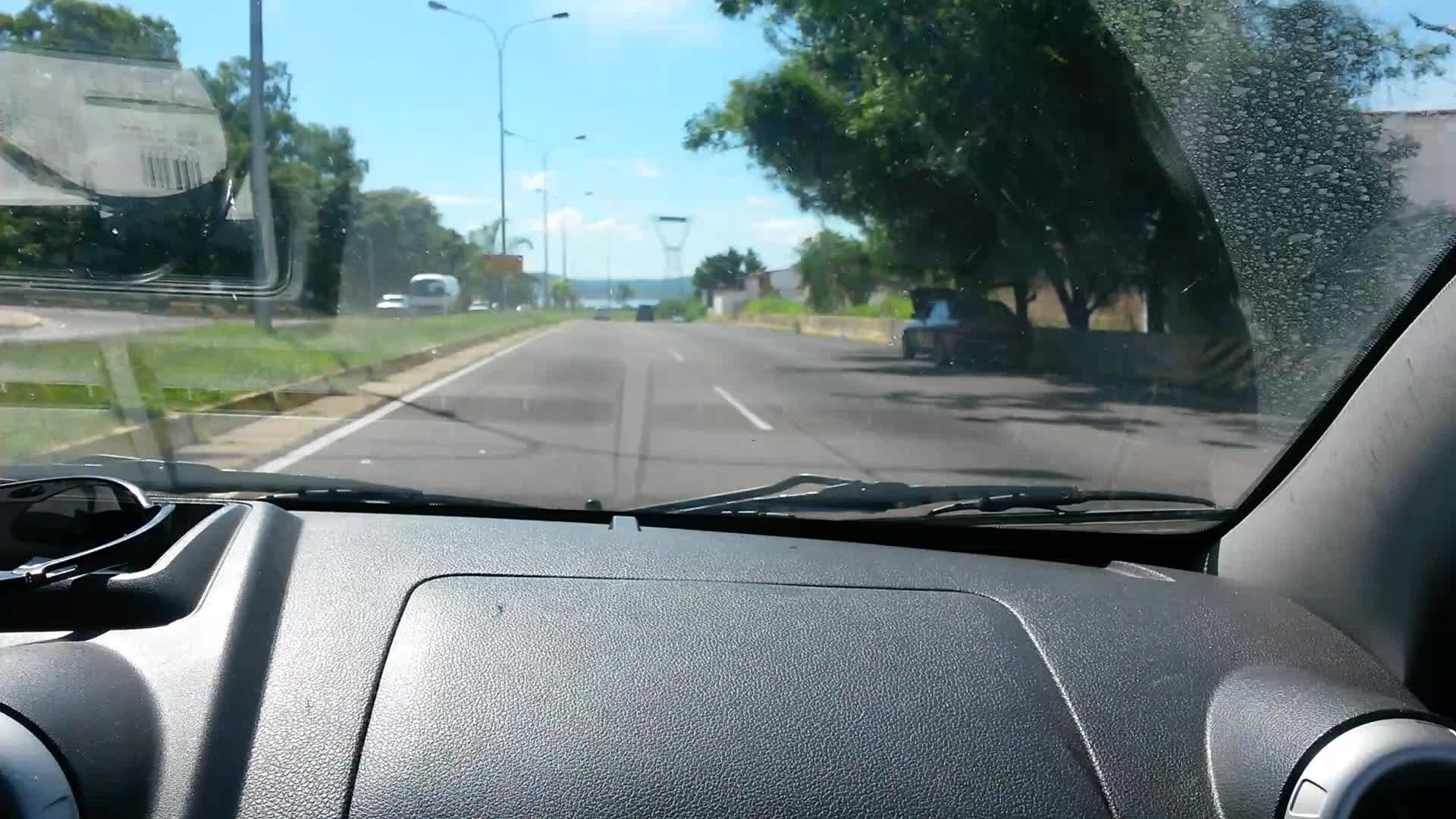A detailed view from within a car shows the vehicle's dashboard at the bottom of the image, offering a glimpse through the windshield onto a bright, sunny day. Outside, the road stretches ahead, with visible street details and a line of trees on the right-hand side. Directly to the right of the observer's vehicle, another car has pulled over to the side of the road under the shade of large trees, with its hood open but no individuals in sight. Across the median, several cars, predominantly white, are headed in the opposite direction. The canopy of the sky above is scattered with fluffy clouds, confirming the clear and sunny weather.